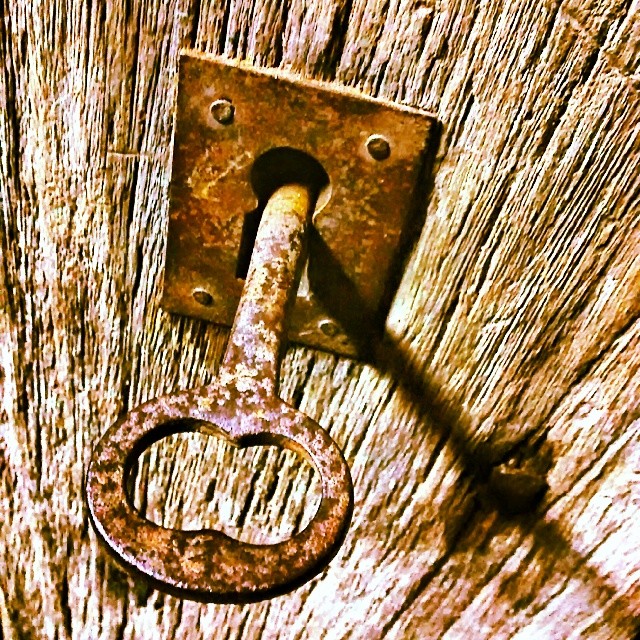This close-up photograph captures an antiquated lock and key set embedded in a heavily worn wooden doorway. The lock, a traditional rectangular metal piece with a distinctive keyhole—round at the top flaring out into a rectangle—is visibly rusted, indicating years of exposure and use. The iron key, featuring a circular ring handle, is currently inserted into the lock and turned, casting a shadow on the weather-beaten door. The door itself is old and splintered, with its surface marked by time and the elements. The image, taken in daylight with sunlight illuminating the scene, suggests a long unmaintained entryway poised to be unlocked, with the inherent tension of whether the key will successfully turn due to the extensive rust.